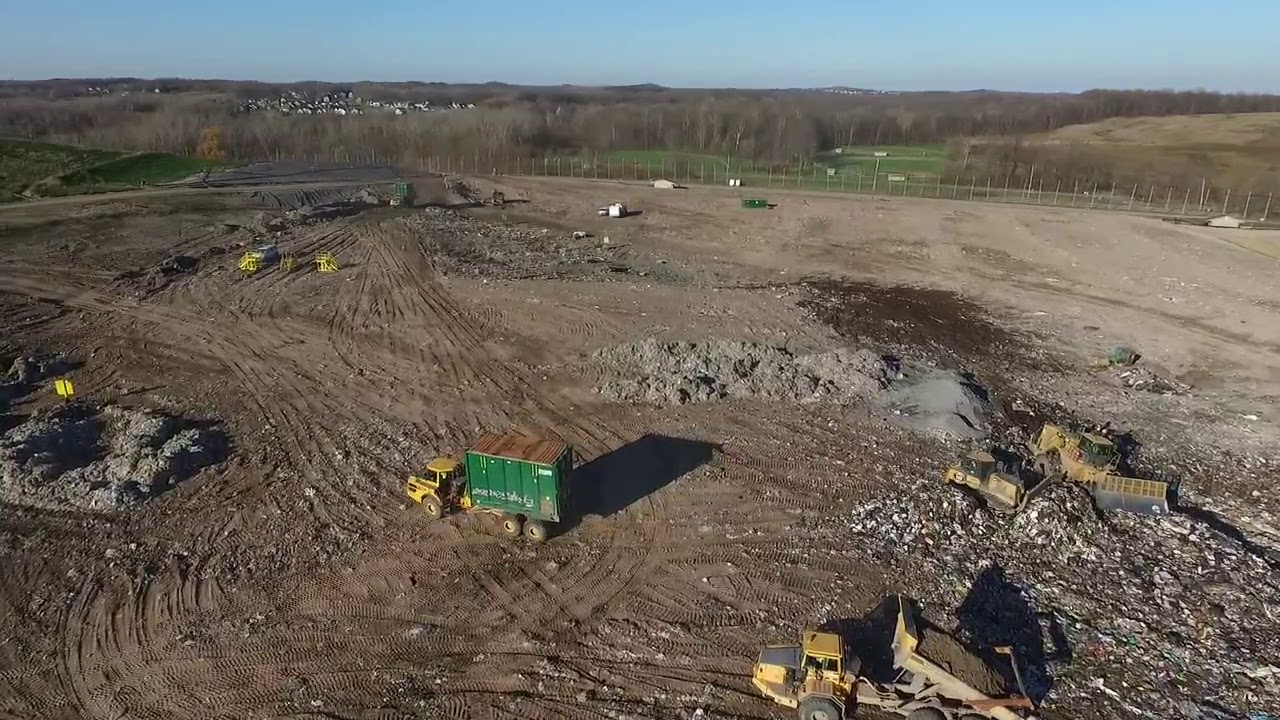The image showcases an aerial view of a dirt-covered site, resembling a construction area or a dumping ground. A number of dump trucks, including one prominently in the foreground, are seen actively unloading debris and soil into various piles of gray and brown shades scattered across the site. Bulldozers can be found pushing these piles into more organized formations. Towards the center, a large green container truck with a yellow cab stands out amidst smaller yellow construction machines in the back left. The entire area is enclosed by a tall, non-solid mesh fence, with visible white poles supporting it. Beyond the fence, to the left rear, a small, manicured green patch is surrounded by bare trees, hinting at the edges of a community or small city in the background. The sky is a clear, vibrant blue, enhancing the overall stark contrast between the barren dirt area and the surrounding hints of civilization.